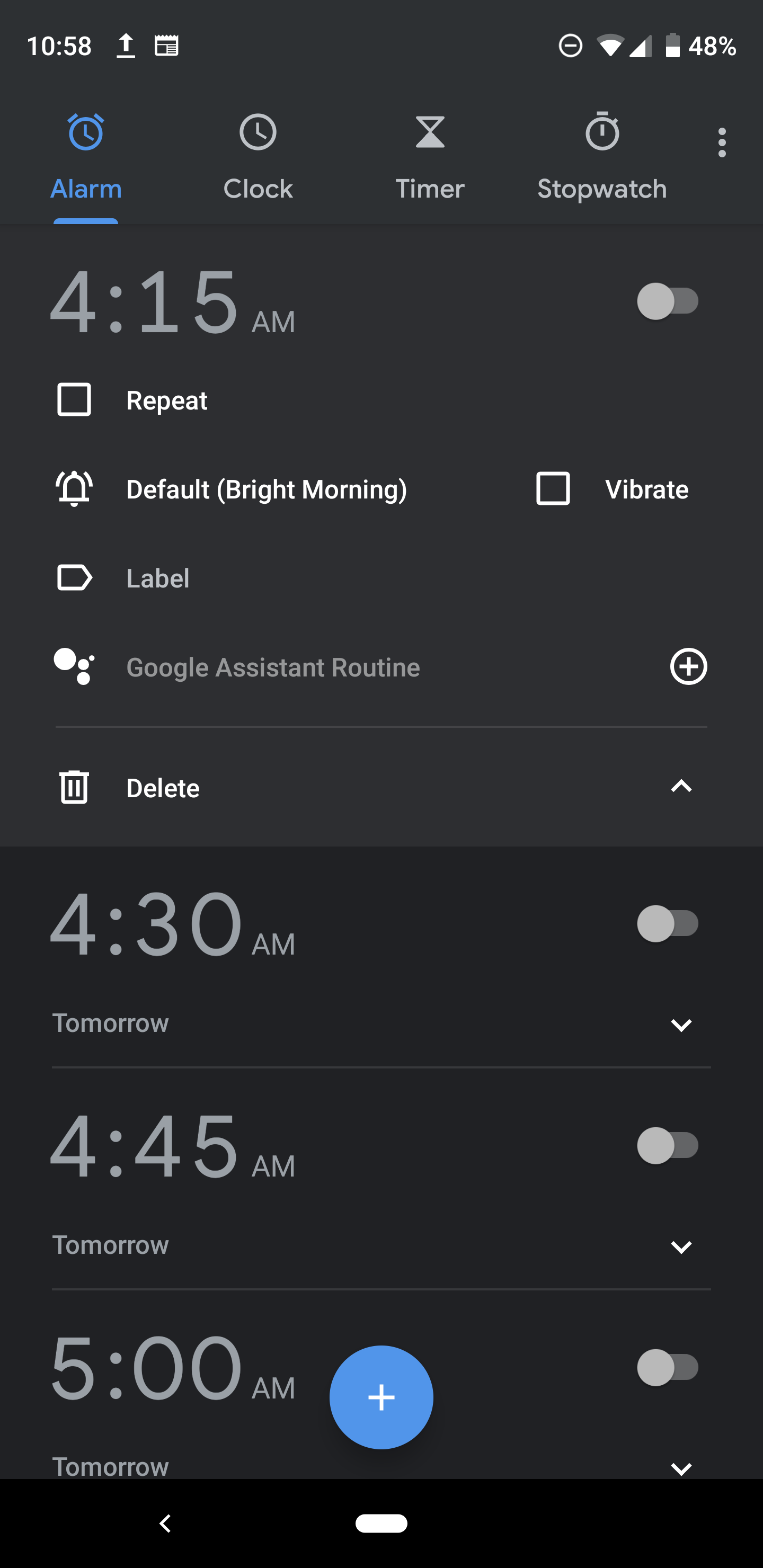A cropped screenshot of a cell phone's alarm settings displayed in night mode, featuring a black background. At the top of the screen, a row of options is visible: Alarm, Clock, Timer, and Stopwatch, with 'Alarm' selected and highlighted in blue, marked by a small blue arrow beneath it. The main portion reveals one active alarm set for 4:15 a.m., accompanied by a toggle switch situated to the right, which is currently in the 'off' position.

Below this alarm time, additional settings are listed: 'Repeat,' which is not specified; 'Alarm default,' set to 'Bright Morning;' and options for 'Label' and 'Google Assistant routine,' both of which appear in gray indicating they are not configured. An unconfigured Google Assistant routine is further highlighted by a plus icon on its right. Below these settings, there is an option labeled 'Delete' for removing the active alarm. Three more alarms are listed underneath this primary alarm for 4:30, 4:45, and 5:00 a.m., but these times are not expanded or detailed further in the screenshot.